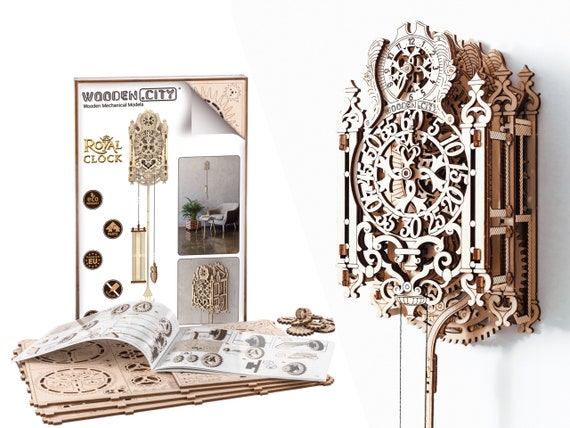The image showcases a highly detailed and ornate 3D wooden grandfather clock, positioned on the right side of the frame. This intricate clock, which may be a puzzle model from Wooden City, displays its internal wooden gears through semi-transparent sides and front, showcasing both its large central clock face and a smaller secondary face at the top. Adjacent to the clock on the left, there is an instruction manual and an informative book displaying various room settings, illustrating how the finished clock would look in different environments. Additionally, the left side of the image reveals the puzzle's numerous components and moving parts, meticulously laid out beneath the instructional booklet. This compelling arrangement not only highlights the craftsmanship of the clock but also serves as a striking advertisement for the assembly process and the final elegant product.